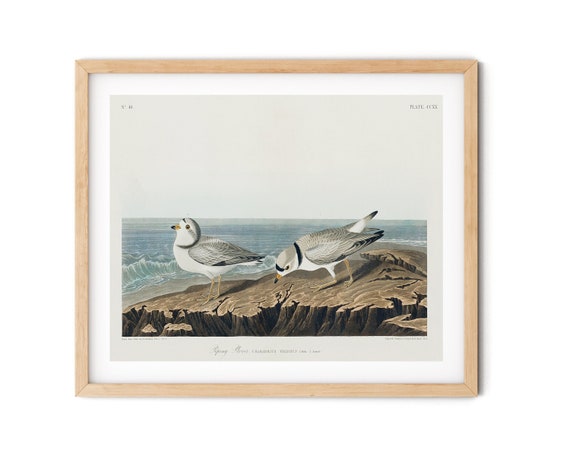This is a framed lithograph-type painting, characterized by very muted colors and enclosed in a light wooden, rectangular frame with a white mat. The artwork features two seagulls, one on the left facing left, and the other with its beak pointed downwards, standing on a rocky outcrop that overlooks a blue-gray ocean. The sea behind them displays gentle waves, while the sky above them is a stark white. The birds, identifiable by their distinct brown necks, gray backs and feathers, white undersides, and short yellow beaks with black tips, appear to be near the water on what could be a small cliff or sand dune. The overall atmosphere of the scene conveys a serene coastal setting. At the top right corner of the painting, there are some black symbols or writing, and beneath the artwork, cursive writing is present but too small to be read. The painting's parchment background enhances its unique and detailed nature.